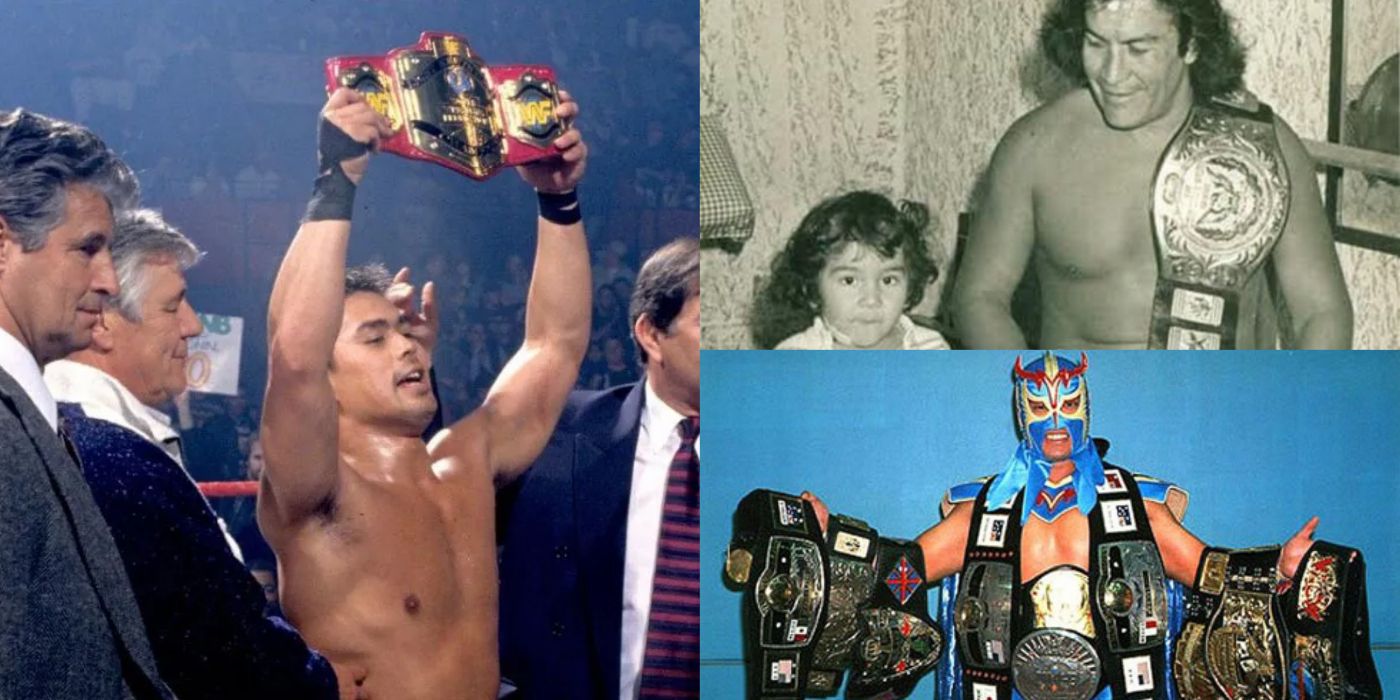This collage contains three photographs that capture the essence of wrestling champions across different eras. On the left, a modern-day bare-chested wrestler is seen jubilantly holding up a large championship belt that is predominantly red with black and gold accents. He is surrounded by three men in suits, suggesting their roles as officials or supporters, while a crowd of spectators in the background add to the celebratory atmosphere.

In the top right, a black-and-white vintage photograph depicts a young boy with curly hair standing next to an older man, likely his father. The man, bare-chested and with long dark hair, gazes down proudly at the boy. A substantial championship belt is draped over the man's shoulder, hinting at his own past glory in the wrestling world.

The bottom right image features a masked wrestler adorned in a colorful lucha libre mask of blue, yellow, and red. This wrestler is covered in numerous championship belts—two over the shoulders, one around the waist, and several draped over outstretched arms. The blue background further highlights the impressive array of belts, emphasizing his dominance and success in the wrestling realm.